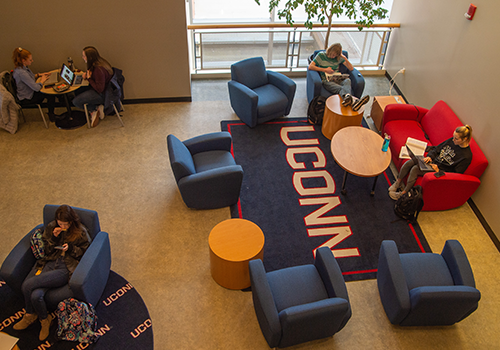The photograph, taken indoors from an overhead perspective, showcases a well-lit study and lounge area at the University of Connecticut, identifiable by the UConn-branded rugs and vibrant decor. The shot captures a cozy, communal space where students are engrossed in their studies and activities. In the center-left, a large UConn rug is surrounded by a cluster of blue chairs, a prominent red couch, and two colorful ottomans. A woman is sitting on the red couch, engaged with her laptop, while another sits nearby in one of the blue chairs, her feet resting on an orange and red ottoman. Towards the center-right and top of the image, a stairwell is visible, suggesting the photograph was taken from the second story or higher. To the far right, two more women are seated at a small table, both using laptops. Below, in the bottom left, another student is absorbed in their phone, snacking while seated on a blue chair atop a round UConn rug. The room has a warm ambiance, reflective of a typical campus environment, perfect for studying and socializing.